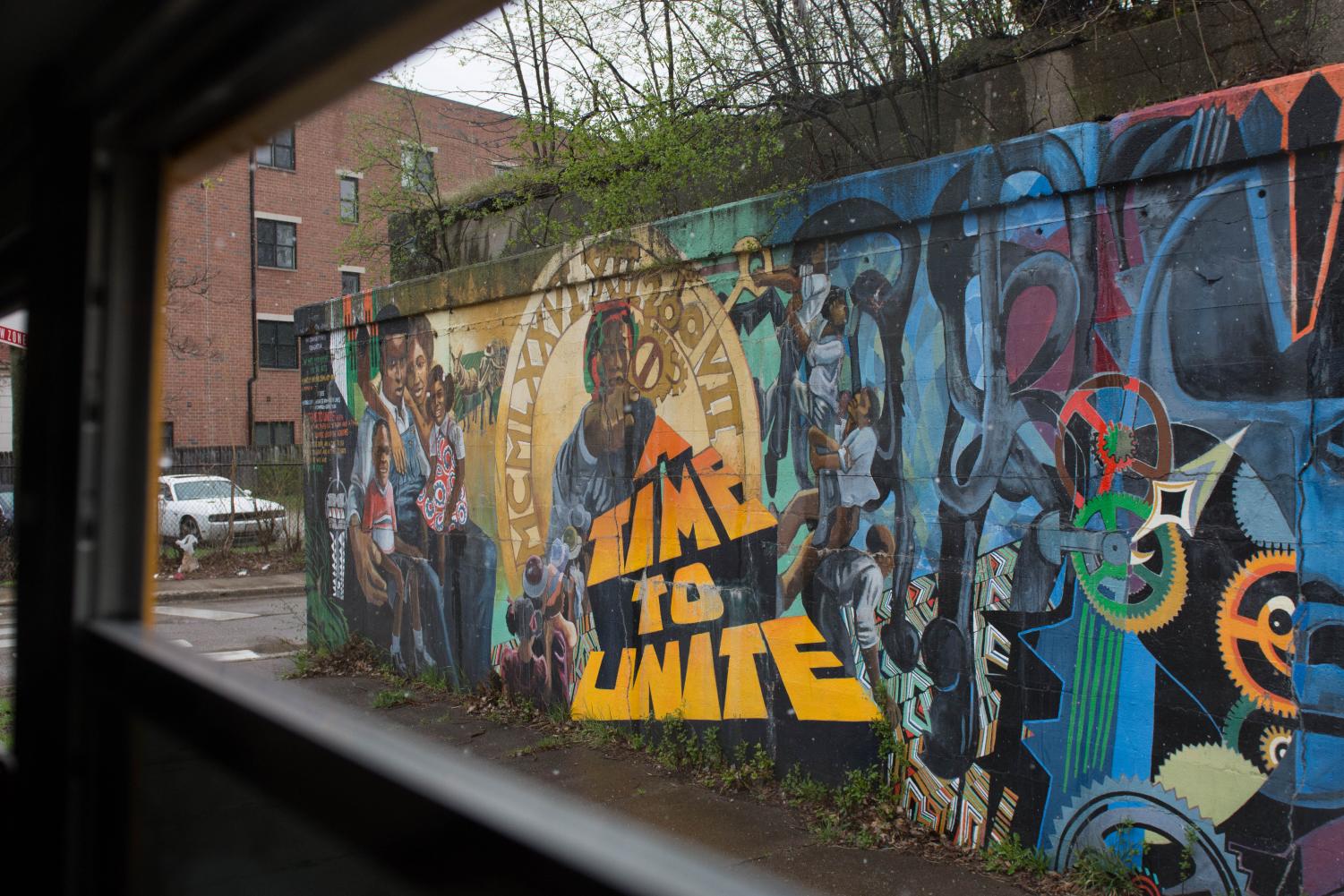This color photograph captures a detailed mural on a dilapidated concrete wall in a rundown neighborhood, taken through an elongated, rectangular window. Dominating the mural is a large, orange-yellow text with black outline that proclaims, "Time to Unite." This message is visually anchored by a central figure of a man surrounded by clock gears and Roman numerals, evoking the internal workings of a watch. The mural is vibrantly colorful, featuring hues of orange, yellow, blue, green, red, and brick red. Various portraits, predominantly of African American individuals, accentuate the theme of unity, including a family scene where a little girl sits on her mother's lap and a boy on his father's lap. On the right, abstract gears in multiple colors can be observed, along with small, unreadable text. The background includes a brick building, a white car parked in what looks like an alleyway, and the tops of green trees, contributing to the scene's overall sense of decay and perseverance.